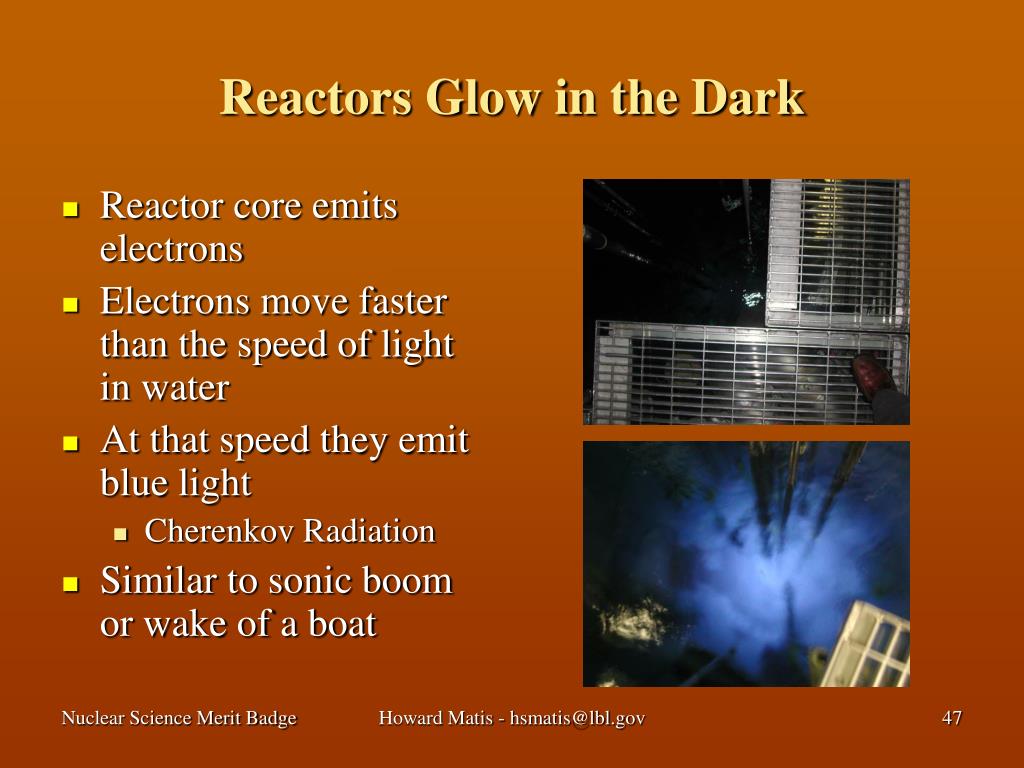This image appears to be a slide from a PowerPoint presentation, generated by Howard Matus for a Nuclear Science Merit Badge. The background features a burnt orange gradient, and the title, displayed in a pale yellow font, reads "Reactors Glow in the Dark." On the left side of the slide, there are bullet points in white text that explain key concepts related to reactor cores:

1. Reactor core emits electrons.
2. Electrons move faster than the speed of light in water.
3. At that speed, they emit blue light. (Cherenkov radiation)
4. Similar to sonic boom or wake of a boat.

Two images on the right side of the slide illustrate these points. The top image shows gray fencing or metal grates, likely part of a reactor core, set against a dark background with indistinct elements, including a small cylindrical object in the bottom right. The bottom image depicts radial blue waves, resembling Cherenkov radiation, emanating from the center against a dark backdrop, with some undefined tan and gray objects in the corners.

At the bottom of the slide, "Nuclear Science Merit Badge" is written in white, along with the contact details "Howard Mattis - H.S. Mattis at LBL.gov" in the middle, and the number "47" in the bottom right corner, indicating the slide number in the presentation.